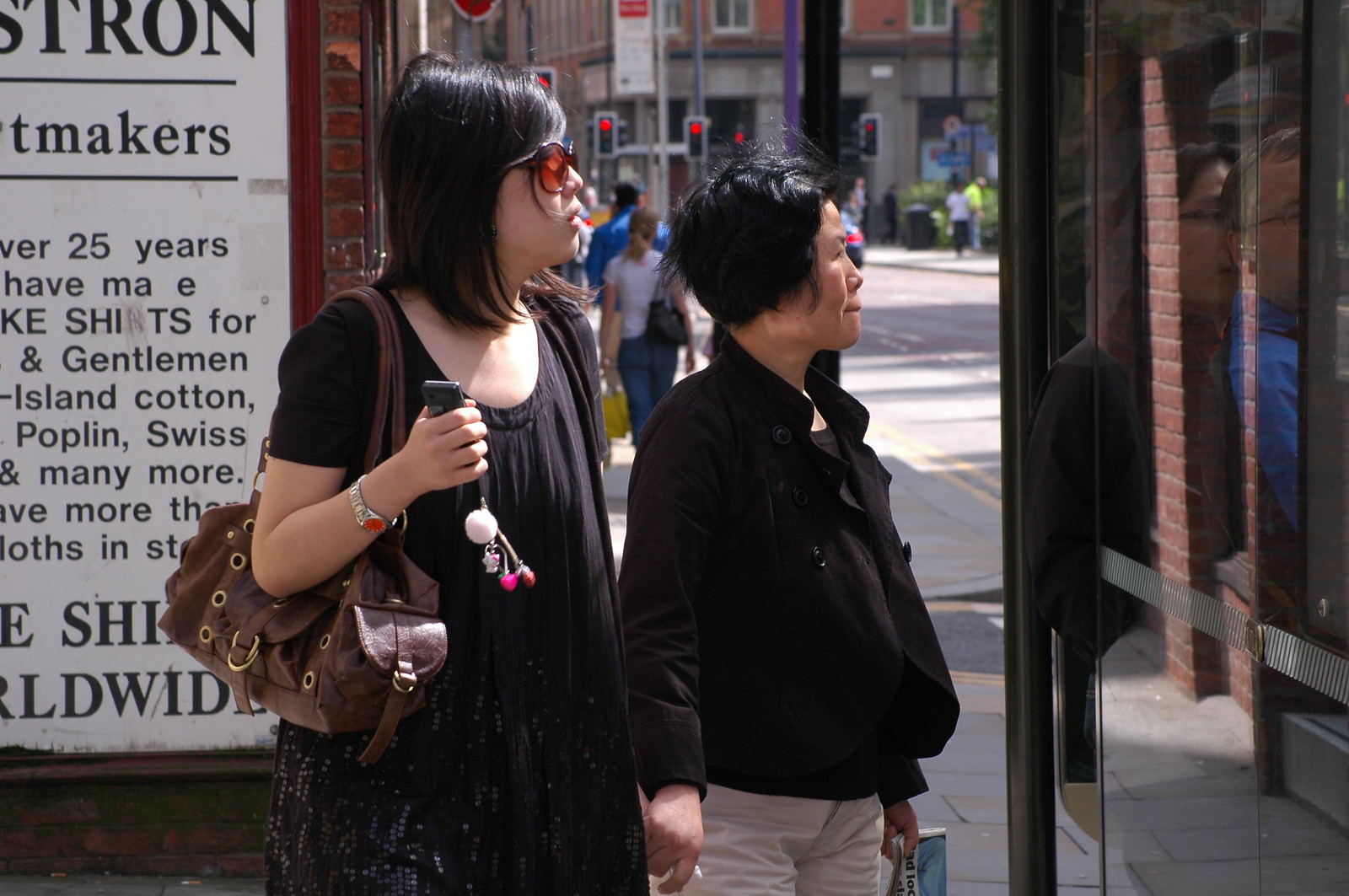This is a detailed photograph of two Asian women standing at what appears to be a bus stop in a bustling city. The background reveals the city's dynamic activity with visible stoplights, people walking around, and various buildings and street signs. Traffic markings are clearly painted on the street. 

The woman on the left is wearing a black dress and sunglasses, has shoulder-length dark hair, and carries a brown purse. She holds a cell phone with dangling items in her right hand and has a watch on her wrist. Behind her, a brick wall features a partially visible poster that reads "25 years" along with some other English words such as "gentlemen," "island cotton," and "Swiss."

Next to her is a shorter Asian woman with short black hair, dressed in a black jacket and white pants. She seems to be grasping the left hand of the woman next to her with her right hand. Both women are looking towards something on their right, possibly a bus or a sign, as their gazes are directed at a black reflective surface, which could be a glass barrier at the bus stop. The scene also shows reflections of buildings and maybe people on the glass surface.